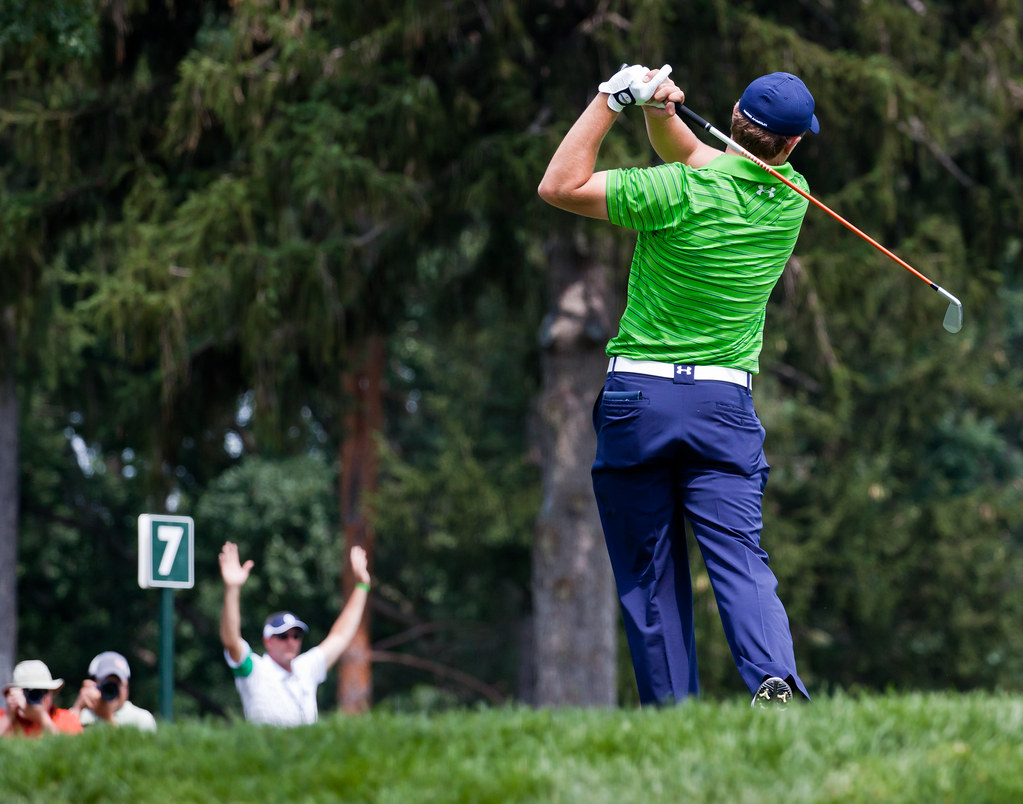The image captures a professional golf game in progress, highlighting a player mid-follow-through. The focus is on a golfer seen from behind, dressed in a light green and black-striped polo shirt, blue pants with a white belt, a white glove on his left hand, and a blue baseball cap. His golf club, which has a black handle, is positioned behind him, suggesting he has just completed a swing. The narrowly focused photograph has a soft blur on the lush green grass in the foreground and the substantial trees in the background. On the left side of the image, two photographers—one in red and one in white, both wearing hats—are captured taking pictures. To their right stands an official, identifiable by his white shirt and a green band over his right bicep, with both arms raised, possibly signaling something. A green pole with a green sign bearing a white number '7' is visible between the photographers and the official, reinforcing the sense of a formal, possibly tournament setting.